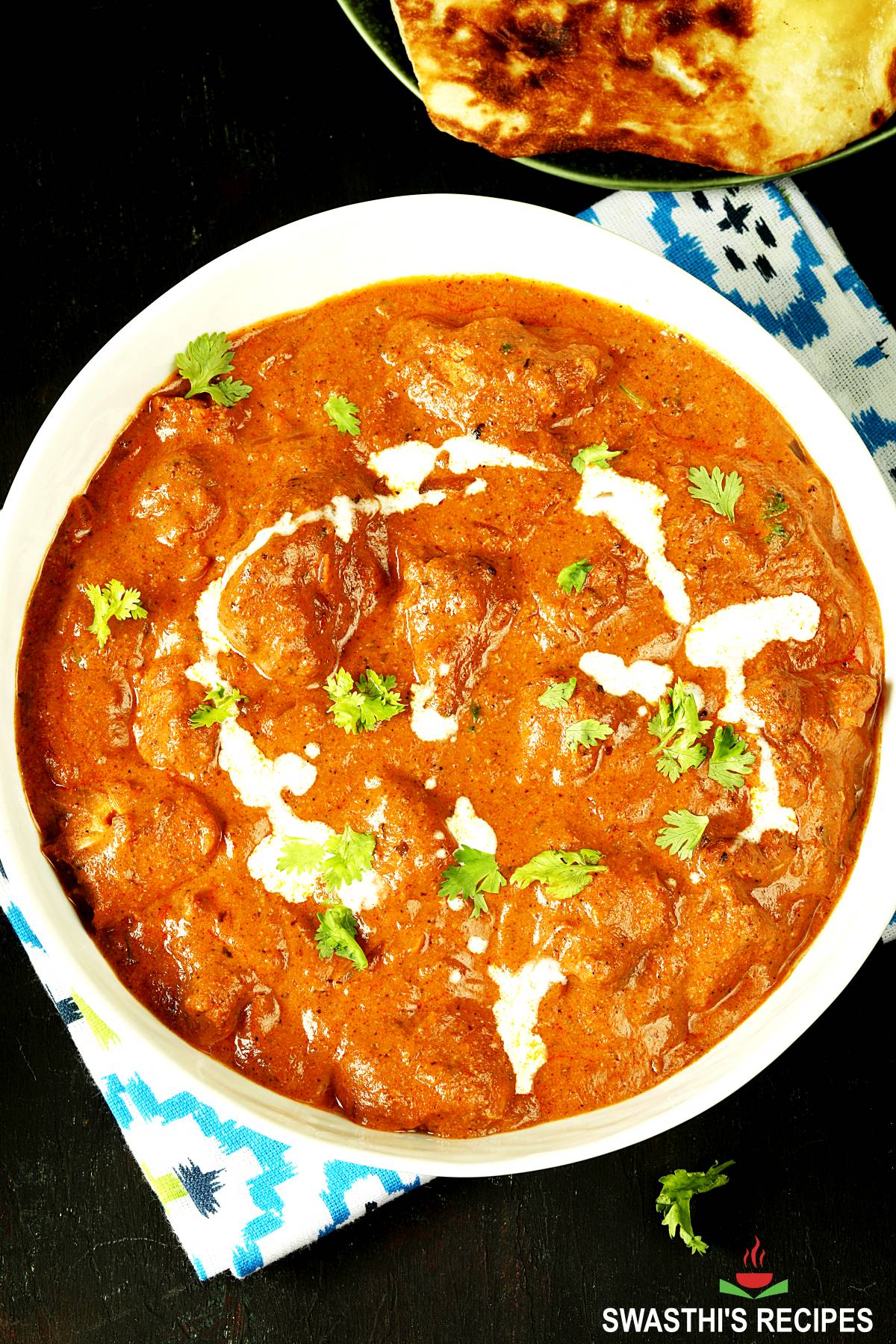The image features a white bowl filled with a dish that appears to be either butter chicken or chicken tikka masala, identifiable by its rich orange tomato-based sauce and chunks of chicken. The dish is garnished with a swirl of cream or yogurt and sprinkled with bits of fresh cilantro. The bowl is placed on a table covered with a black surface and a blue and white cloth. At the bottom right of the image, there's text in white font that reads "Swasti's Recipes," accompanied by an icon of a steaming bowl with red steam swirls above it. In the upper right corner of the image, part of another bowl is visible, appearing to contain a piece of flatbread, likely naan. The overall setting suggests a well-prepared meal ready to be enjoyed.